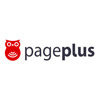The image showcases a zoomed-in view of a logo with a white background, which might suggest it has a transparent background in its original format, such as a PNG. Central to the image is the logo text "page plus" and an adjacent simplistic owl emblem.

On the left side, the owl logo is rendered in red. The owl's design is minimalistic, with two white circles for eyes and a single dot for the beak. The owl's body consists of three inverted, Wi-Fi-like symbols, also in white, giving it a distinctive, streamlined appearance.

To the right, the logo text "page plus" is presented in dark gray. The word "page" is in regular, unbolded font, while "plus" is in bold, maintaining the same dark gray color. Notably, the typography features specific details: the "L" in "plus" is curved, and the "G" in "page" has an open, unlooped structure. This combination of elements creates a clean and modern aesthetic for the brand.